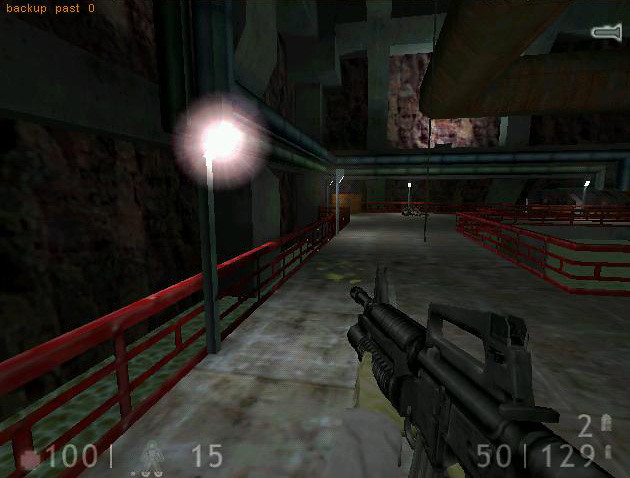The image is a screen grab from a first-person shooter video game. Dominating the lower right-hand side of the screen is the player’s perspective, showcasing an M4 carbine rifle. While the actual player remains unseen, the first-person viewpoint confirms the shooter genre. Positioned clearly on the bottom right corner, the HUD displays ammunition details: 50 bullets currently available out of a total capacity of 129, accompanied by the number '2', likely indicating grenades. On the opposite side, the left bottom corner, there is a health indicator showing '100/100' health, possibly the maximum, and a smaller '15', suggesting body armor, both depicted next to an icon of a person.

The setting is an underground environment, akin to a bunker or an industrial cave structure, characterized by a blend of raw rock surfaces and extensive metal infrastructure. Metal beams and red rusty railings line the dark concrete pathway which is sporadically illuminated by overhead lights. Ductwork, piping, and vents run along the walls, enhancing the gritty, industrial atmosphere. Additional on-screen text includes "back up" and "past" in gold or orange letters in the upper left-hand corner, along with a cryptic series of numbers in white font scattered around the interface.